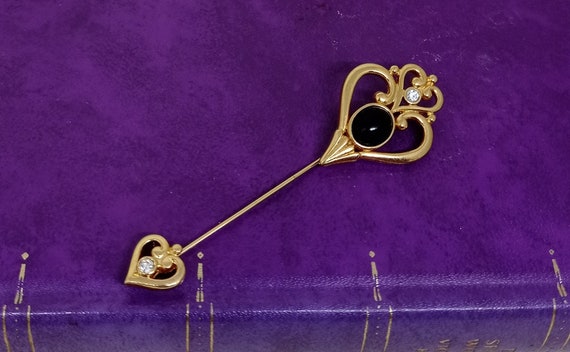This is a color photograph featuring an antique gold pin resting on a royal purple, leather-bound book. The pin itself is intricately designed, resembling the style of an antique key. It has a long, thin base, suggesting it might be a hat pin. The focal decorative element is a larger heart at the top, adorned with an onyx cabochon at its center and a small diamond in a smaller heart above it. This larger heart is surrounded by detailed gold scrolling. The lower part of the pin features a smaller heart with a slight scroll at the top and a small diamond enclosed within it. The pin's gold color harmonizes with the gold lines and embellishments on the spine of the book, which is partially visible in the photograph. The spine features two central gold lines, two more on the left and right sides, and some barely legible letters, including an "S" and a "W." The photograph emphasizes the pin as the central element against the luxurious backdrop of the purple book.